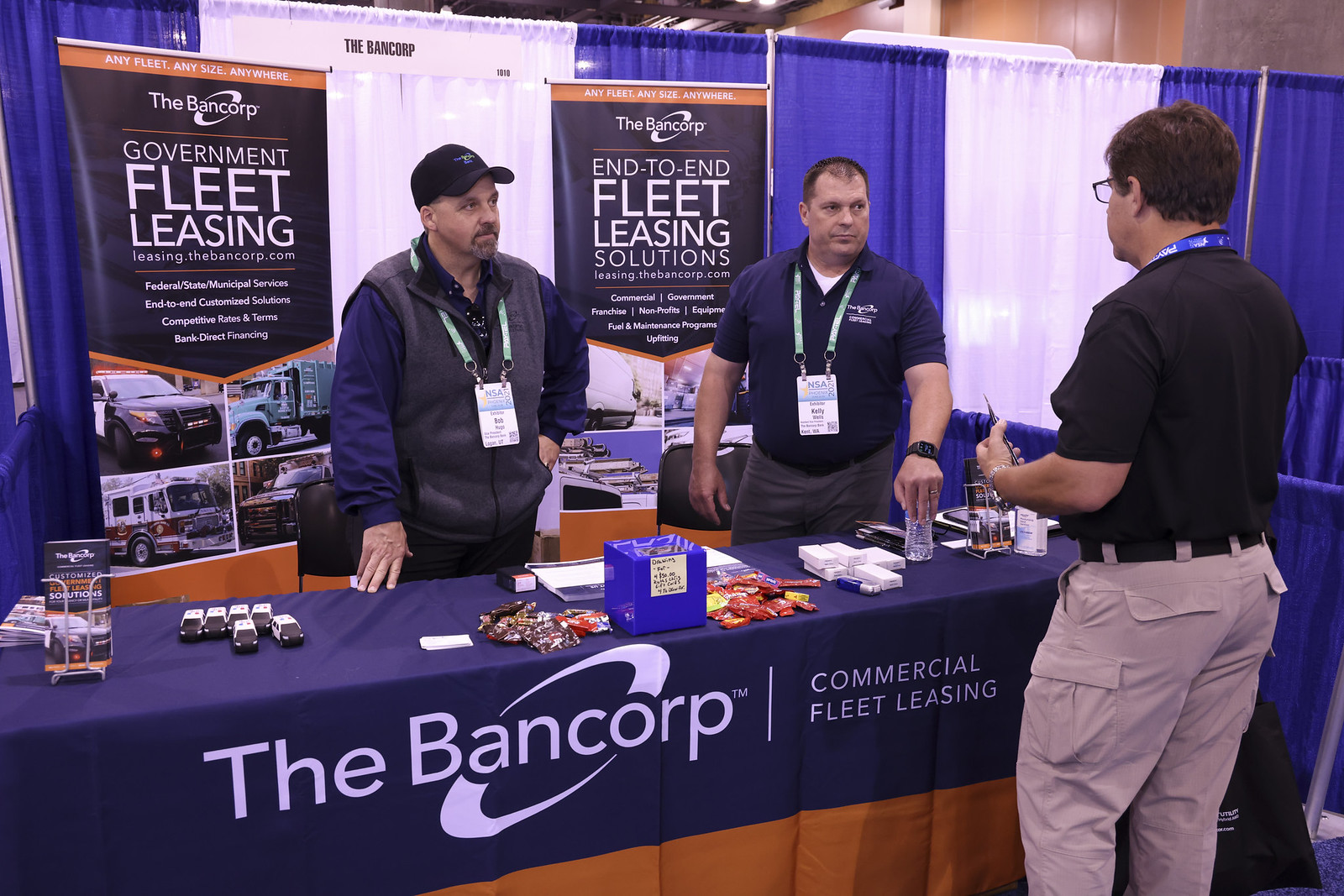This photo captures a bustling scene at a travel-related trade show or convention. Central to the image is a booth from Bancorp Commercial Fleet Leasing, featuring two middle-aged men behind a table covered with a blue tablecloth displaying their logo. The man on the right wears a blue polo, while the man on the left is donned in a blue baseball cap, black vest, and blue long-sleeved shirt. Both wear green lanyards and name tags indicating they're part of the event, possibly NSA 2021. They’re conversing with a man in a black polo, blue lanyard, and beige cargo pants, standing in front of the table. Behind the booth, a blue and white curtain serves as a backdrop for two prominent signs: "Government Fleet Leasing" and "End-to-End Fleet Leasing Solutions," which feature images of cars and trucks. The table is laden with brochures, miniature toy cars, various giveaways, and candy, making for an inviting and informative display.